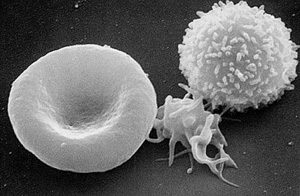This detailed microscopic image captures a close-up view of various microorganisms against a stark black background speckled with tiny white dots. On the left, there is a prominent, round shape with a characteristic central indentation, resembling a white-hued red blood cell. Moving towards the center, there is a distinct formation of long, white strands clumped together, seemingly connecting the cell-like structures. In the upper right corner, another spherical organism is visible, adorned with small, spike-like protrusions, giving it a textured appearance reminiscent of shredded coconut. The overall palette of the image is limited to black, white, and gray, emphasizing the intricate details of the cellular forms and the empty expanse surrounding them.